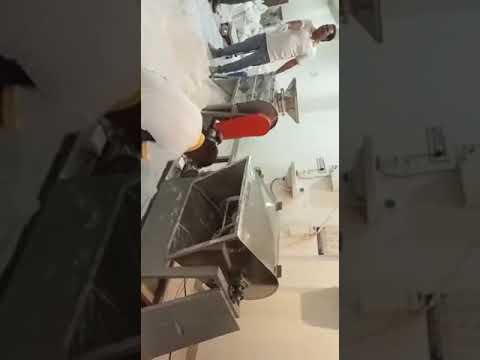The image shows a scene inside a large, enclosed room with three men engaged in what appears to be construction or maintenance work. The orientation of the image is tilted sideways, adding to the disjointed yet detailed view of the activities within. The men are dressed uniformly in white t-shirts paired with jeans, and notably, one man is wearing gloves. Their faces are not visible as they are cropped out or turned away. One man is crouching with his back turned to the camera, another is carrying a bucket, and the third man is partially visible up to his stomach.

Scattered throughout the room are numerous off-white cloth bags featuring green, red, or black and red writing. These bags appear to be filled with materials, contributing to the workspace's cluttered appearance. The room itself has a white floor, which looks like it might be undergoing some patching or flooring work.

Additionally, there is a gray mechanical object with a black hole visible in the scene, though this machinery is mostly cropped out and hard to identify. You can also spot a desk or table among the bags, further emphasizing that the room is being used for some form of manual labor. The left and right sides of the photo are blurry and devoid of color, presenting a stark contrast to the central, more detailed part of the image.